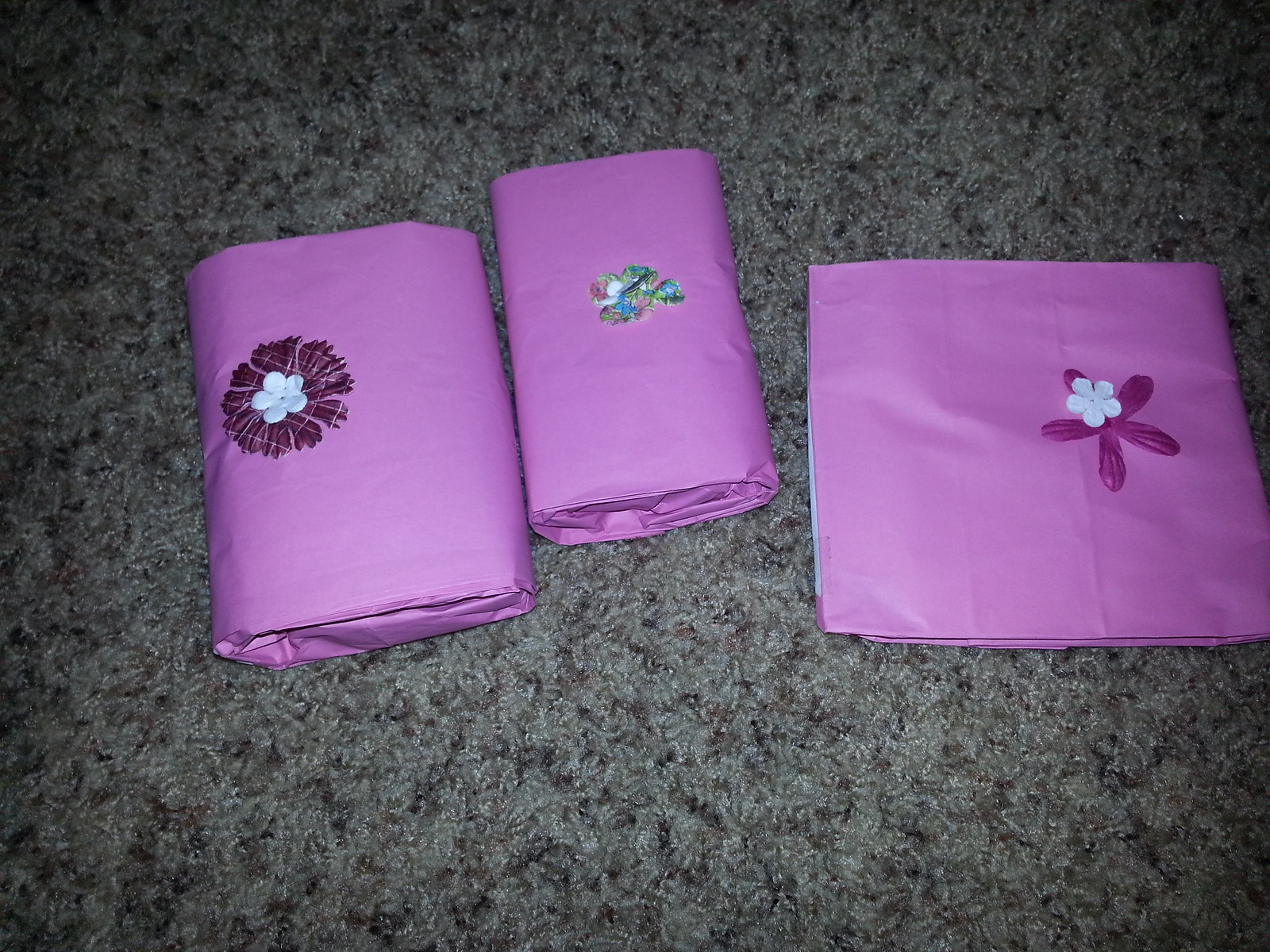This photograph captures a dimly lit scene featuring a dark gray carpet with black and brown speckles, providing a stark contrast to the vibrant items placed upon it. Central to the image are three neatly wrapped gifts, all adorned in a bright purple wrapping paper. On the left, a rectangular gift is wrapped in lavender-colored paper accented with a striking burgundy and gold checker pattern and topped with a white five-petaled flower. The middle gift, equally rectangular, features a prominent blue and green flower-shaped sticker with intricate, colorful details. Positioned to the right is a square package, adorned with a dark purple five-leaf flower underlined by another white five-petal flower. The thoughtful arrangement of the gifts, with two on the left and one on the right, creates a balanced, visually appealing composition on the moody carpet backdrop.